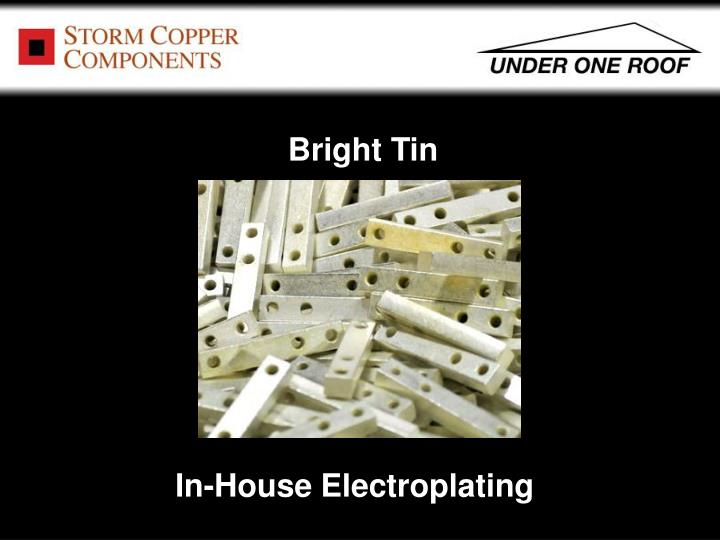The image appears to be a digitally designed advertisement, possibly for use in a magazine or newspaper, highlighting the services of Storm Copper Components. On the top left, the company's name, "Storm Copper Components," is displayed in red letters beside a logo consisting of a red square enclosing a smaller black square. On the top right, there is a right-skewed triangle with the tagline "Under One Roof" positioned beneath it. Below this, the main visual element features a large black rectangular background framing a clear photograph of metallic components. These components are silver rectangular blocks with three holes—two on one side and one on the other—suggesting their use for connections involving screws or wires. Above and below the photo, white text reads "Bright Tin" and "In-house Electroplating," respectively, indicating specialized plating services offered by the company.